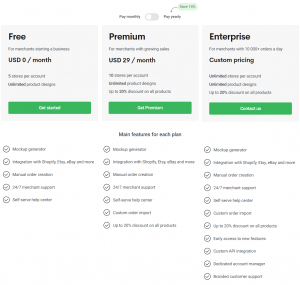The image features a comparison chart with three gray boxes aligned horizontally at the top. Each box represents a different pricing tier for a service.

- **Left Box (Free Plan):**
  - **Header**: "Free"
  - **Price**: "USD $0 a month"
  - **Button**: A green "Get Started" button at the bottom of the box.

- **Middle Box (Premium Plan):**
  - **Header**: "Premium" in bold black letters
  - **Price**: "USD $29 a month"
  - **Details**: Contains a block of text that is too small and blurry to read.
  - **Button**: A green button at the bottom.

- **Right Box (Enterprise Plan):**
  - **Header**: "Enterprise" in bold black letters
  - **Price**: "Custom Pricing"
  - **Details**: Contains a block of text that is too small and blurry to read.
  - **Button**: A green button at the bottom.

At the very top between these three boxes is a toggle bar, positioned to the left.

Below the boxes, there's a line of text centered on the image. Directly under this text are three columns (left, middle, and right), each listing features associated with the plans. Each line in these columns has a circle with a checkmark beside it, though the specific text next to the checkmarks is not readable.